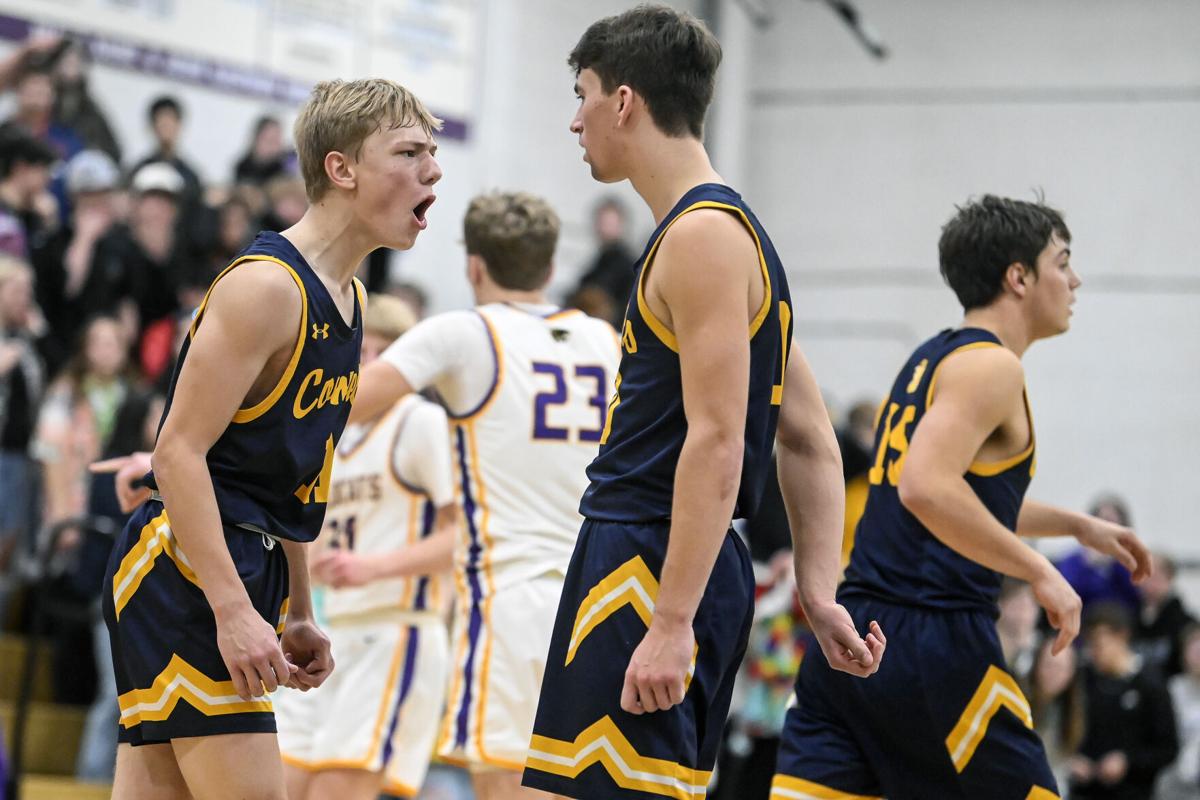In this image, a spirited high school basketball game is taking place in an indoor gymnasium, evidenced by the white walls and absence of any visible windows. Central to the scene are three boys clad in dark blue jerseys with gold fringes and accents, likely from the same team. The player on the left, a blonde boy with short hair, appears to be yelling towards his taller, brown-haired teammate in the middle. The third teammate, positioned further to the right, is captured mid-action, moving away from his peers. Despite their animated interaction, there's no basketball or hoop in sight, adding a layer of ambiguity to the exact moment captured.

In the background, a competing team can be seen wearing predominantly white jerseys with blue, gold, and purple stripes. Among them, both a player facing away and another partially turned towards the camera are vaguely discernible. Adding to the vibrant atmosphere, a sizable crowd is present, seated on bleachers primarily along the left side of the image, observing the ongoing game. The overall scene is a dynamic snapshot of youthful energy and competition.